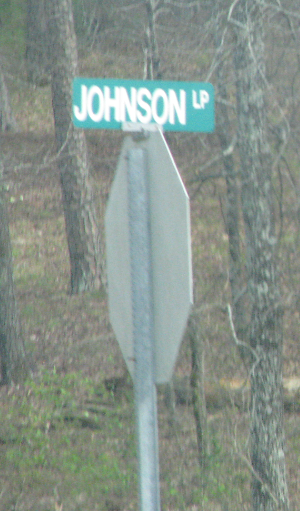The image captures a densely wooded landscape, dominated by an abundance of trees with firm, textured bark. Numerous branches extend from these trees, adding to the thick foliage. The ground is primarily composed of dirt, interspersed with patches of green moss that lend it a slightly verdant appearance. Prominently positioned in the foreground is a stop sign affixed to a metal pole. Above the stop sign is a green street sign indicating "Texas Johnson LP." To the right, more branches extend from the trees, contributing to the dense, wooded ambiance. The overall focus of the image appears slightly blurry, likely emphasizing the scene's natural, rustic quality.